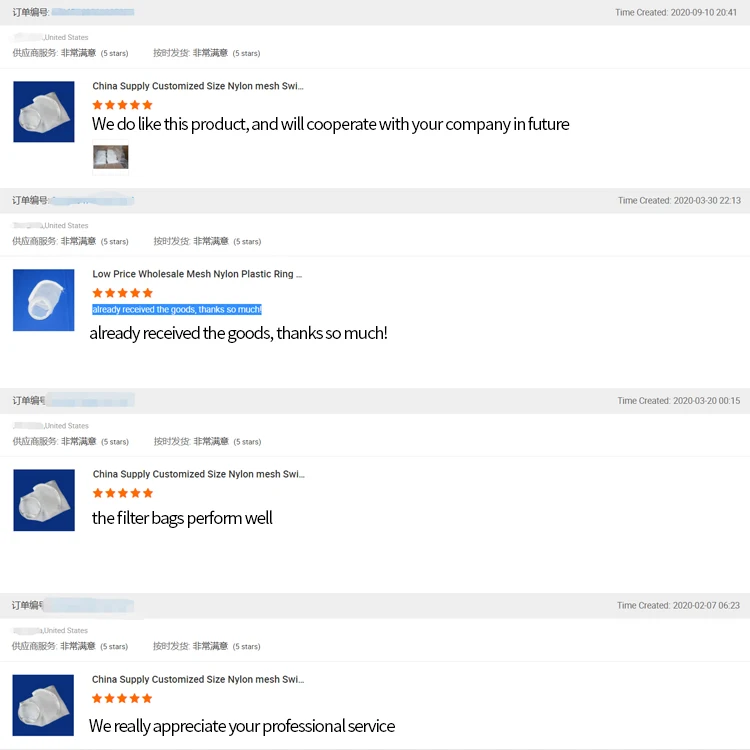A screenshot of a website is displayed featuring content predominantly in kanji. The top section, marked by a gray background, records the creation time as "2020-09-10 20:41." Below this, the text "United States" is visible with some text crossed out before it, followed by kanji characters and the phrase "five stars." Repeatedly, kanji and "five stars" (in English) indicate high ratings.

Beneath, the text "China supply custom size nylon mesh SWI..." is shown, accompanied by a product endorsement: "Do we like this product? Yes, we do like this product and will cooperate with your company in the future." A photograph of a white mask on a blue background is featured next to this text.

Further down, kanji characters and a blurred section are observed, with text reiterating "United States," kanji, and "five stars." It reads: "Low price wholesale mesh nylon plastic ring... already received the goods, thank you so much," highlighted in blue with white font. 

Following this, the exact same message is repeated: "Already received the goods, thank you so much." 

The next review again mentions "United States" with some crossed-out text, accompanied by kanji and "five stars." The text reads: "China supply custom size nylon mesh SWI..." praising the product: "The filter bag performed well." The same image of the white mask on the blue background appears recurrently throughout these reviews.